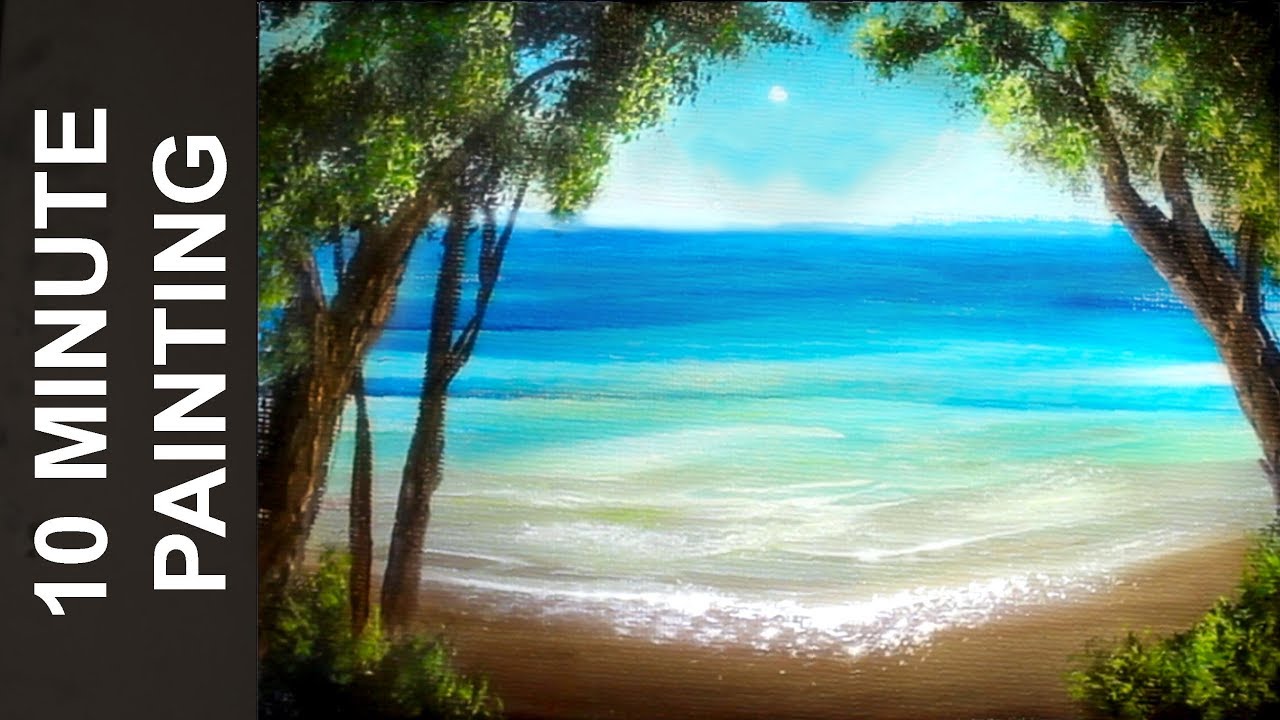This is a detailed painting of a beach scene, created in oil paints and capturing a vivid and layered depiction of nature. The painting is framed in landscape orientation, showcasing the shoreline from a unique perspective between two large trees on either side. These trees, with their rich foliage, form a natural arch over the scene, guiding the viewer’s eyes towards the beach. At the bottom left and right corners, there are shrubs adding more depth and greenery to the piece. 

The beach itself features white waves gently lapping onto the sandy shore, with the water transitioning from a light aqua near the shore to a darker blue further out. The sky above is a clear blue, dotted with low white clouds on the horizon and a small white sun or moon positioned overhead, enhancing the serene atmosphere. 

On the left-hand side of the painting, there is a black vertical rectangle with white text that reads "10-minute painting," adding an element of graphic design to the artwork. The light reflection in the painting is particularly striking, bringing brightness to the foreground and casting gentle shadows towards the back, highlighting the artist's skill in depicting light and depth.